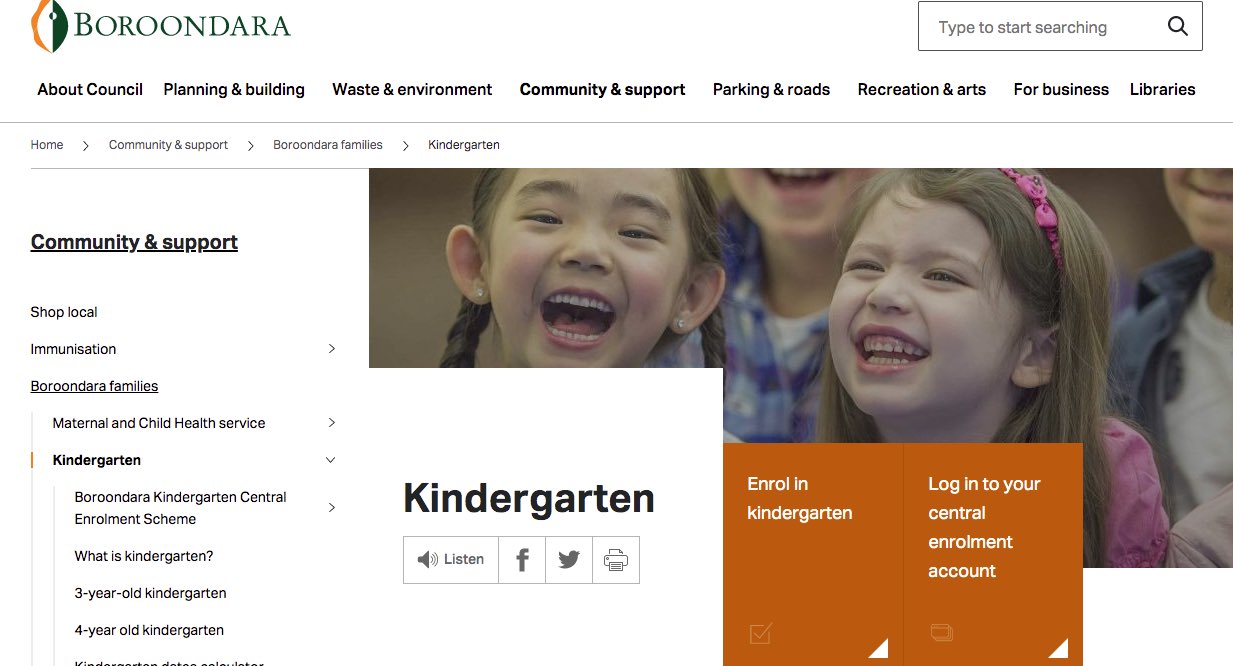The image features a website layout with a predominantly white background. At the top of the page, the heading "Boron Dara" is prominently displayed in bold text. On the right-hand side, there is a search field labeled "Type to start searching." Below the header, a series of navigation links are listed under various categories including "Council," "Planning and Building," "Waste and Environment," "Community and Support," "Parking and Roads," "Recreation and Arts," "For Business," and "Libraries."

The viewer’s eye is drawn to the "Community and Support" section, which includes subcategories like "Shop Local," "Immunizations," "Boron Dara Families," "Maternal and Child Health Service," and "Kindergarten." The text "Boron Dara Families" and "Kindergarten" are particularly highlighted in very bold black type, indicating their importance. The phrase "Kindergarten Central Enrollment Scheme" is also prominently displayed within this section.

Moving to the right side of the page, there is a cheerful photograph of two little girls. One girl has her hair styled in braids while the other has her hair down, adorned with a pink headband that matches her dress. Both girls are laughing, exuding a sense of joy and friendship. Beneath the picture, the word "Kindergarten" appears.

Adjacent to this image is an orange box containing the call-to-action to "Enroll in Kindergarten" and instructions to "Log in to your central enrollment account." The overall design and content of the page clearly aim to guide users towards kindergarten enrollment, making the process as straightforward as possible.